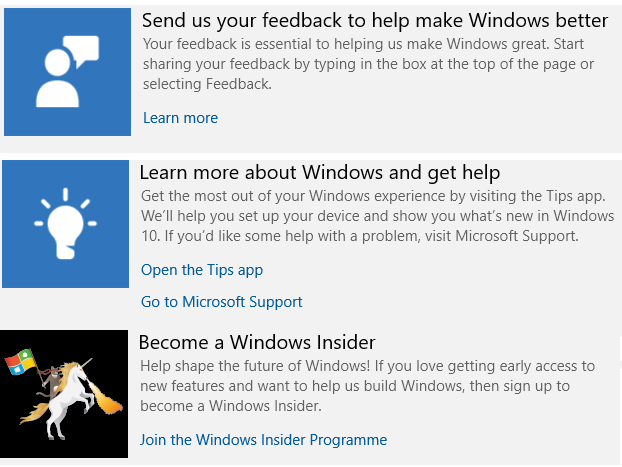A digital display interface, divided into three distinct sections, provides various Windows-related resources and programs. 

1. **User Feedback Invitation**: 
   - **Visual Elements**: This section features a minimalist white silhouette of a person against a black background. To the right of the figure, there is a gray message icon.
   - **Text Content**: The header reads, "Send us your feedback to help make Windows better." Below it, a detailed description emphasizes the importance of user feedback in enhancing Windows. Users are encouraged to start sharing their thoughts by typing in a box at the top of the page or by selecting the feedback option. A clickable "Learn more" link in blue offers additional information.

2. **Windows Tips and Support**:
   - **Visual Elements**: This section displays a graphic of a light bulb emitting rays of light.
   - **Text Content**: The headline states, "Learn more about Windows and get help." The description invites users to maximize their Windows experience by visiting the Tips app, which aids in device setup and showcases new Windows 10 features. For troubleshooting, users are directed to Microsoft support. The options "Open the tips app" and "Go to Microsoft support" are presented as clickable blue links.

3. **Windows Insider Program**:
   - **Visual Elements**: A stylized, cartoon-like image depicts a white horse rearing on its hind legs, ridden by a person waving a multicolored flag in green, red, blue, and yellow.
   - **Text Content**: The header reads, "Become a Windows Insider." A narrative follows, encouraging passionate users who enjoy early access to new features and want to contribute to Windows development to join the Windows Insider Program. It ends with a prompt to "Join the Windows Insider Program" as a clickable invitation for participation.

This interface collectively fosters user engagement through feedback, provides educational resources, and invites users to participate in the ongoing development of Windows.